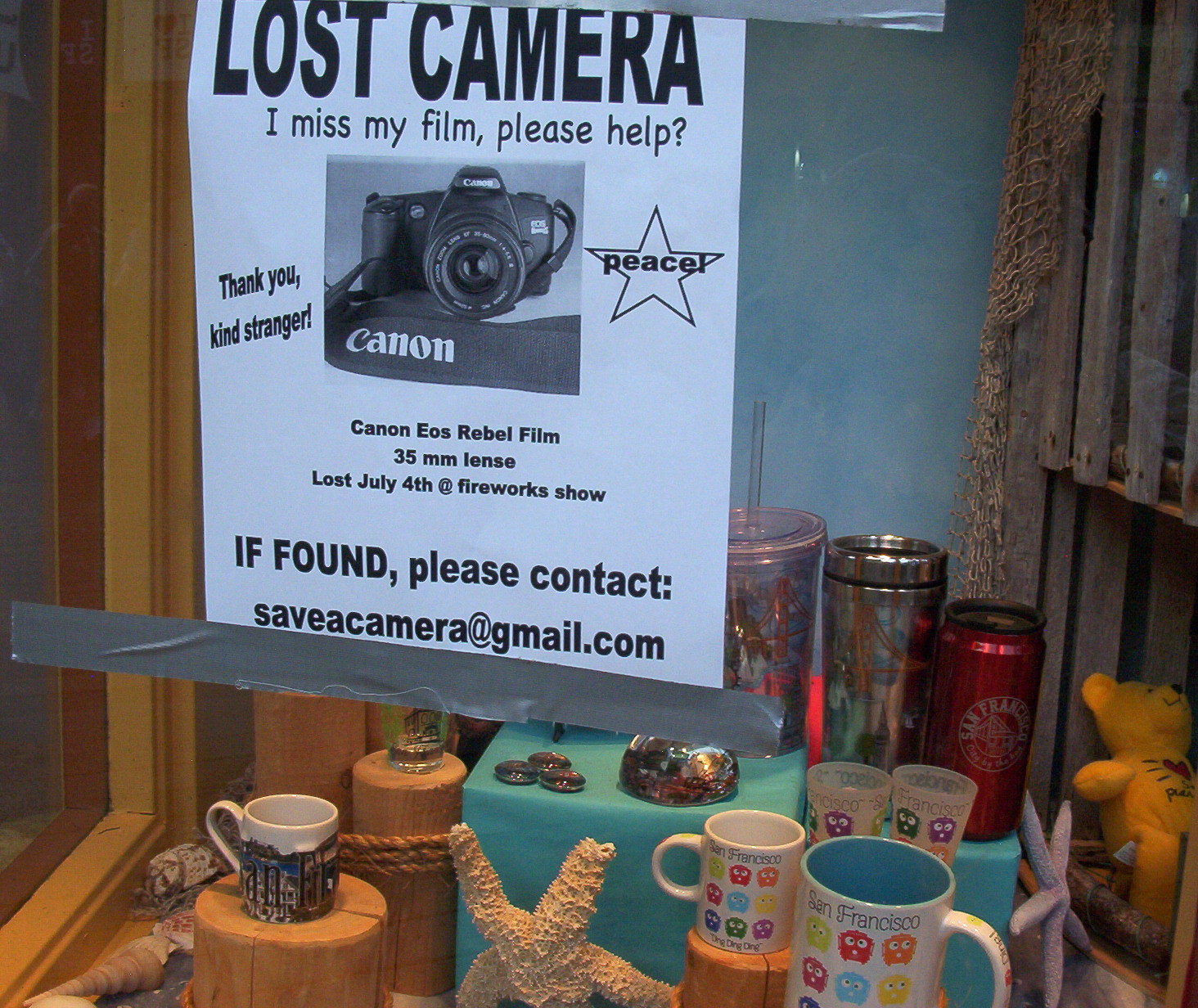This image shows a store display window with a sign taped to the glass using strips of silver masking tape at the top and bottom. The sign takes up the upper quadrant of the image and has black text on a white background. It reads: "Lost camera. I missed my film. Please help. Thank you, kind stranger." There is a picture of a Canon camera with the word "Canon" underneath it, and a star with the word "peace" in the middle. Beneath the image, the text continues: "Canon EOS Rebel film, 35mm lens. Lost July 4th at Fireworks show. If found, please contact SaveACamera@gmail.com." Behind the window display, you can see various items including water bottles, coffee mugs with "San Francisco" and ghost designs, tumbler cups, starfish, shells, and what appears to be a type of jeweled stone. There is also an orange teddy bear in the lower right-hand corner and a little blue wall in the background.